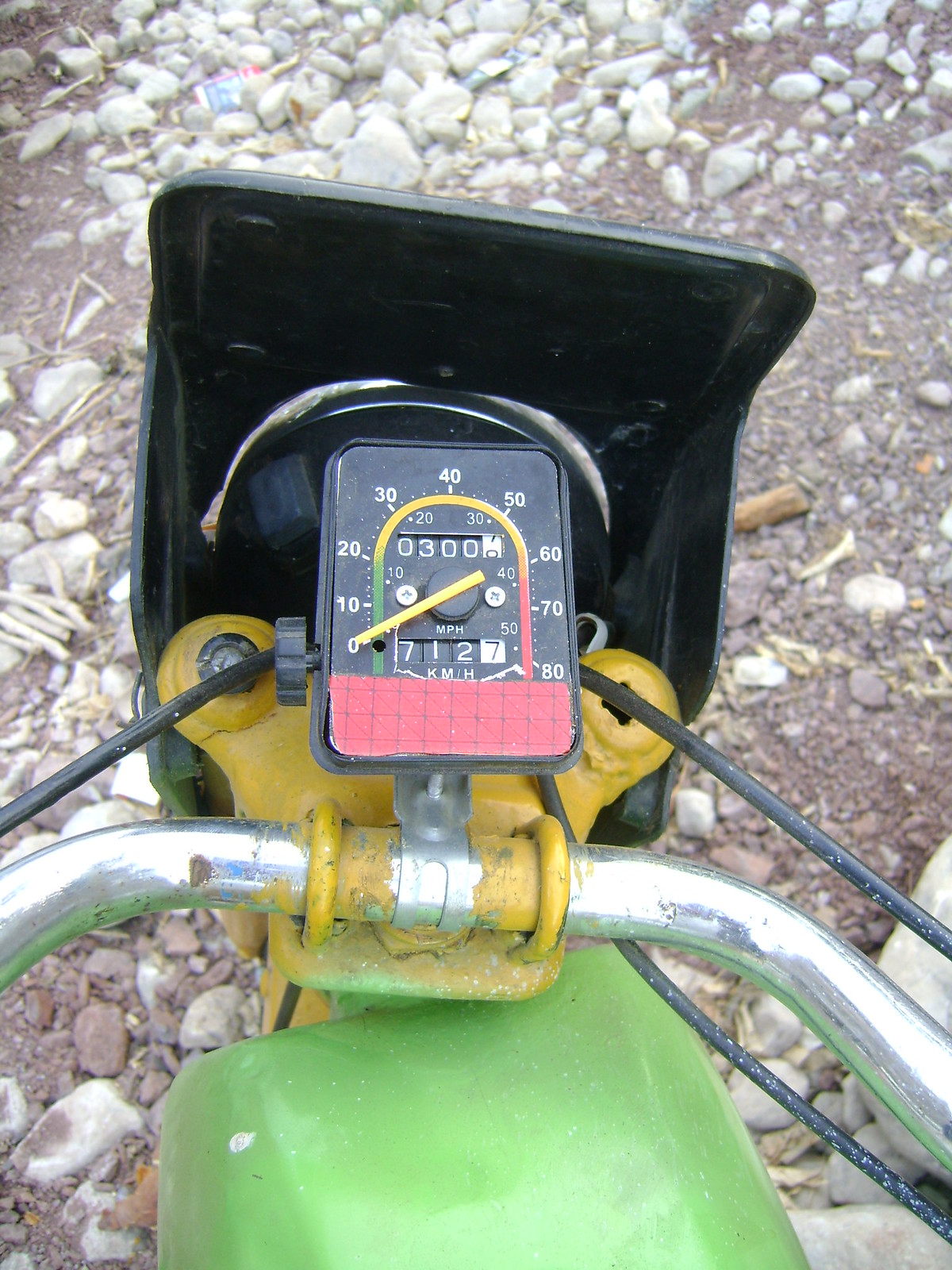The image depicts a cluttered scene on a ground covered with numerous small white rocks and scattered pieces of wood. Near the upper center-left, there is an indistinct object displaying a blend of blue, purple, and pink hues. Adjacent to it is a nearly black or dark green item intertwined with elements of silver.

Dominating the center of the image is a rectangular device outlined in black. The top three-quarters of this device have a dark background accentuated with numbers and lines that vary in thickness. An arch-shaped spectrum begins from the left in green, transitions to yellow, and finally turns pink as it curves downward on the right. Within the yellow portion of the arch is a counter displaying "0300." A yellow hand, presumably intended to move along the scale, sits atop the dial.

Below the yellow portion are the inscriptions "MPH" and "712" against a black backdrop, followed by a "7" set on a white background. The bottom of the device has a pink section with a yellow element featuring two bulb-like structures connected by metallic components and appearing to have tubes emanating from behind.

The device is held in place by a metal framework that curves. Visible adjacent to this metal framework and device are glimpses of the ground with rocks and dirt. A light green object stretches to the bottom of the image, contributing to the complex assortment of items.